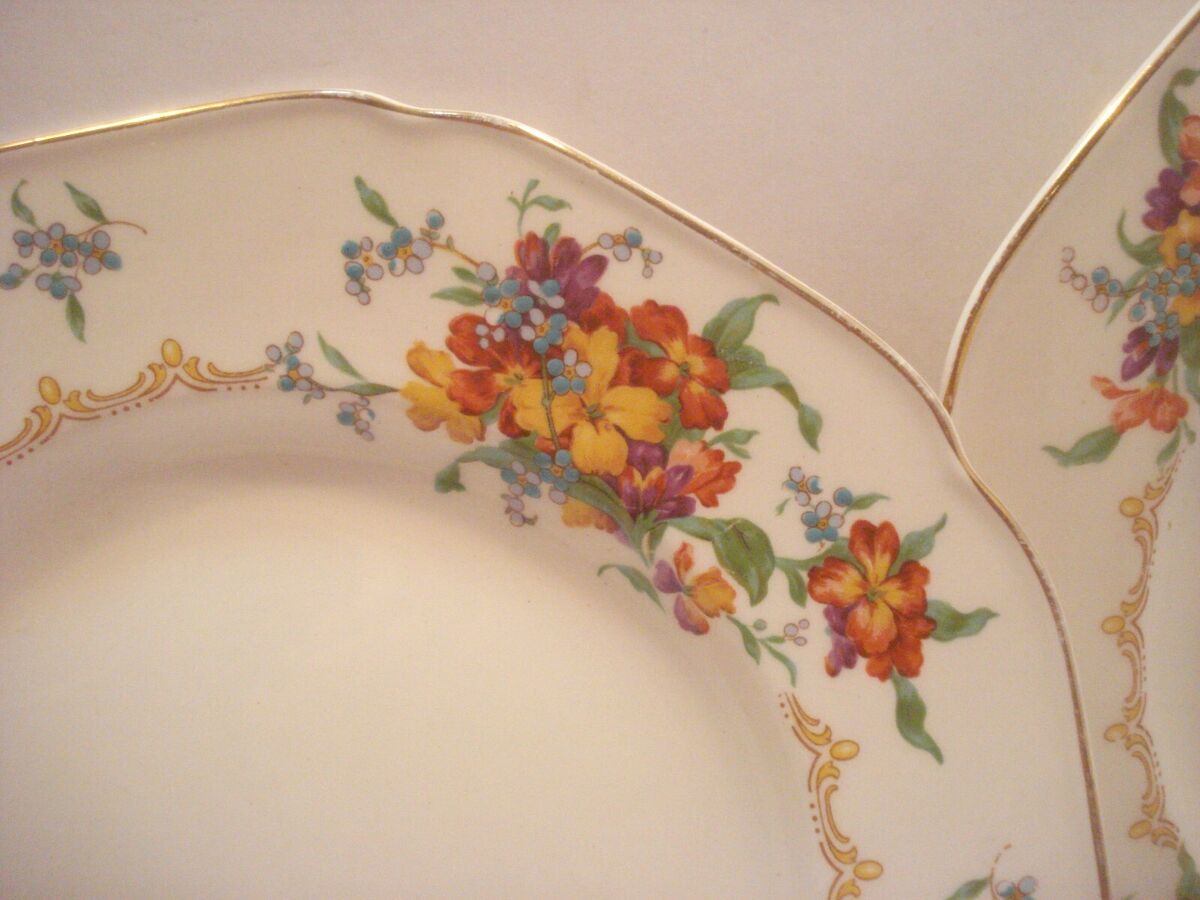This is a detailed close-up photo showcasing the intricate design of two fine china plates. The plates, only partially visible in the image, are adorned with a bouquet-like floral pattern featuring red, yellow, purple, and small blue flowers, all interspersed with green leaves. The center of each plate is white, while the rims are elegantly detailed with gold foil lines and scalloped edges, giving them a luxurious appeal. These plates, seemingly part of the same set, are the type typically reserved for display rather than everyday use, resting on a plain, light-colored table.